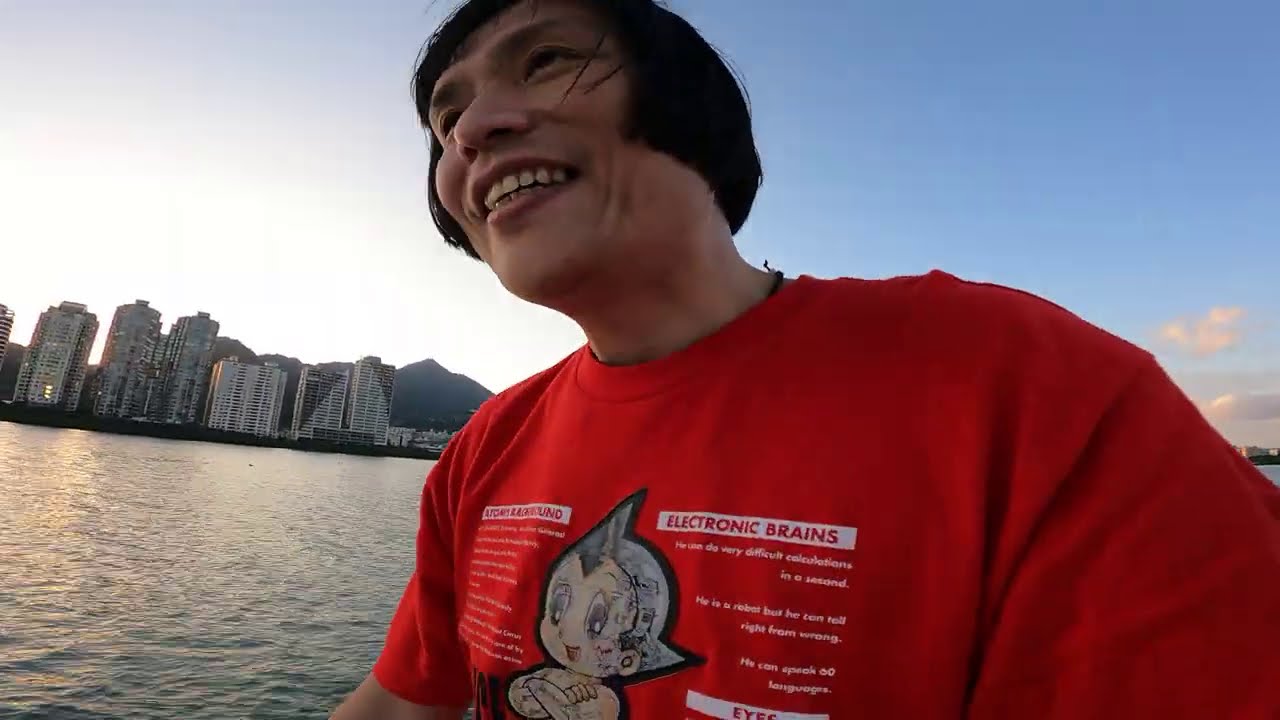The image captures a woman with very short pixie-cut black hair, wearing a red shirt featuring a character, likely Astro Boy, and some writing including "electronic brains." She is smiling and looking off to the left side of the frame. The background reveals a scenic view with a large body of water that reflects the sunlight, suggesting it might be a lake or sea. On the opposite shore of the water, there's a sprawling cityscape with numerous high-rise skyscrapers concentrated more on the left side and smaller buildings to the right. Beyond the city, a tall mountain range stretches across the horizon under a clear, blue sky. The photo appears to be taken either from a boat or a small dock, as indicated by the proximity to the water and the natural outdoor lighting.